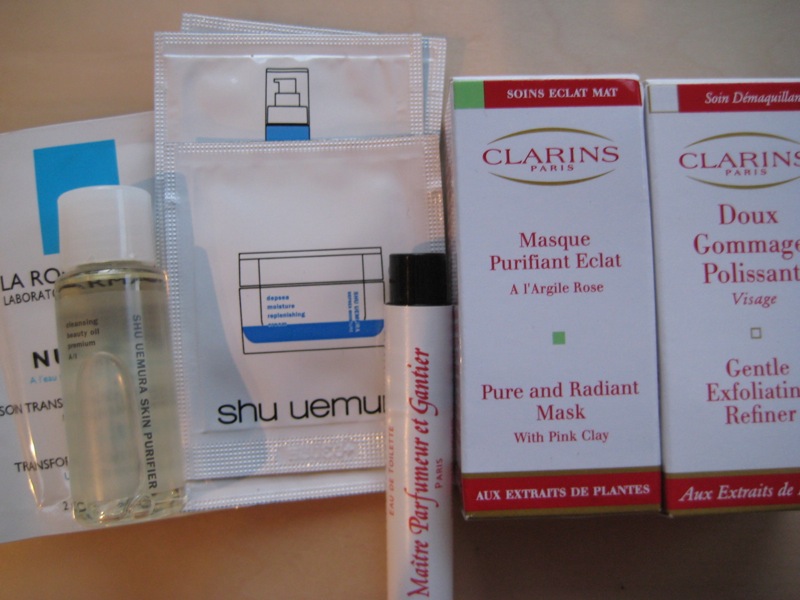This image showcases a variety of facial cosmetics neatly arranged. On the right, there are two boxed products from Clarins. The first box, labeled in red on a white background, reads "Clarins Paris Masque Purifiant Éclat" indicating it is a Pure and Radiant Mask with Pink Clay. The second box next to it bears the label "Clarins Paris Doux Gommage Polissant," describing it as a Gentle Exfoliating Refiner.

To the left of these boxes is a cylindrical container with a black cap and white body, featuring red lettering indicating it is a type of perfume. 

Further to the left, there are several plastic packets from the cosmetic brand Shu Uemura, although the contents of these packets are not specified.

Continuing leftward, there is a small, clear plastic bottle containing a semi-transparent lotion, capped with white. Behind this lotion bottle, a white plastic packet with blue markings from La Roche-Posay is partially visible, adding another layer of skincare variety to the collection.